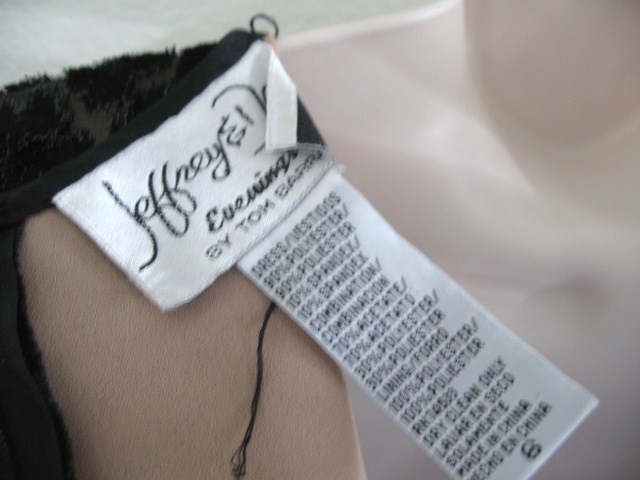The photograph is in a landscape format, featuring a background that is indistinct but predominantly white and appears to be either a bag or a table with a wavy texture. In the bottom left corner, there is an item that looks like either a fur boot or glove. The interior of this item is primarily dark brown and fluffy, while the exterior has a varied pattern in shades of white, grey, and brown, with a thin strip of brown fluff extending downward.

Attached to this item is a product tag displaying the brand name, "Jeffreys Euphoria by Tom Barry," written in a calligraphy-like, scribbly font on a white label. A longer product tag is also present, detailing the fabric composition and care instructions: "Dress 90% polyester, 10% spandex combination, 70% acetate, 30% polyester lining, 100% polyester. Dry clean only." These tags suggest the item requires specific care and provide a meticulous breakdown of the materials used.